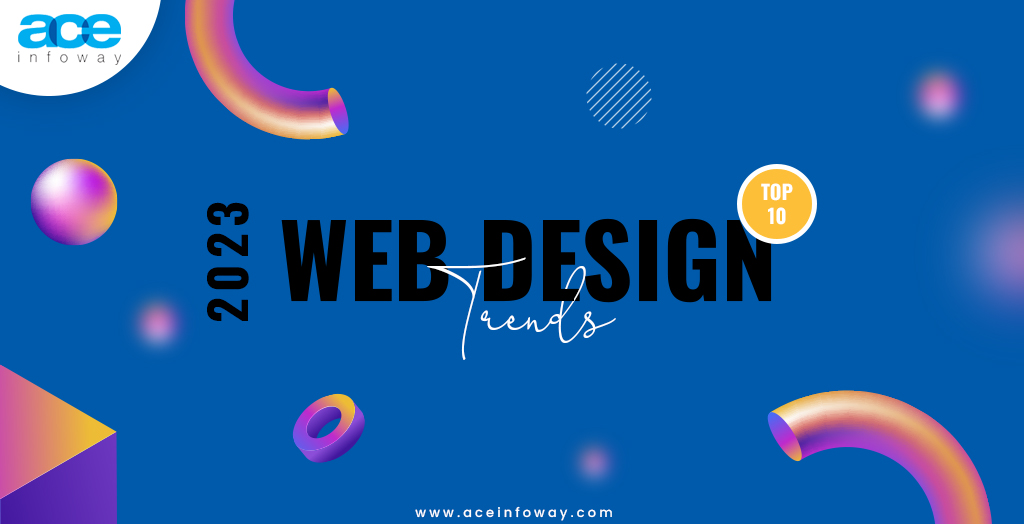This image is a detailed poster or banner for a website, showcasing "2023 Web Design Trends." The background is a medium blue color adorned with vector geometric shapes including spheres, cubes, discs resembling washers, and tubes, featuring gradients of orange, purple, and shades of pink. At the top left corner, within a yellow semicircle, it reads "AceInfoWay." Prominently in the center, large block letters spell out "2023 Web Design," with "Trends" elegantly superimposed in a white cursive font. There is also a yellow circle near the word "Design" containing "Top 10" in white letters. At the very bottom, the website address "www.aceinfoway.com" is displayed. The design features a mix of tube-like and circular vectors that add a dynamic and modern aesthetic to the overall image.